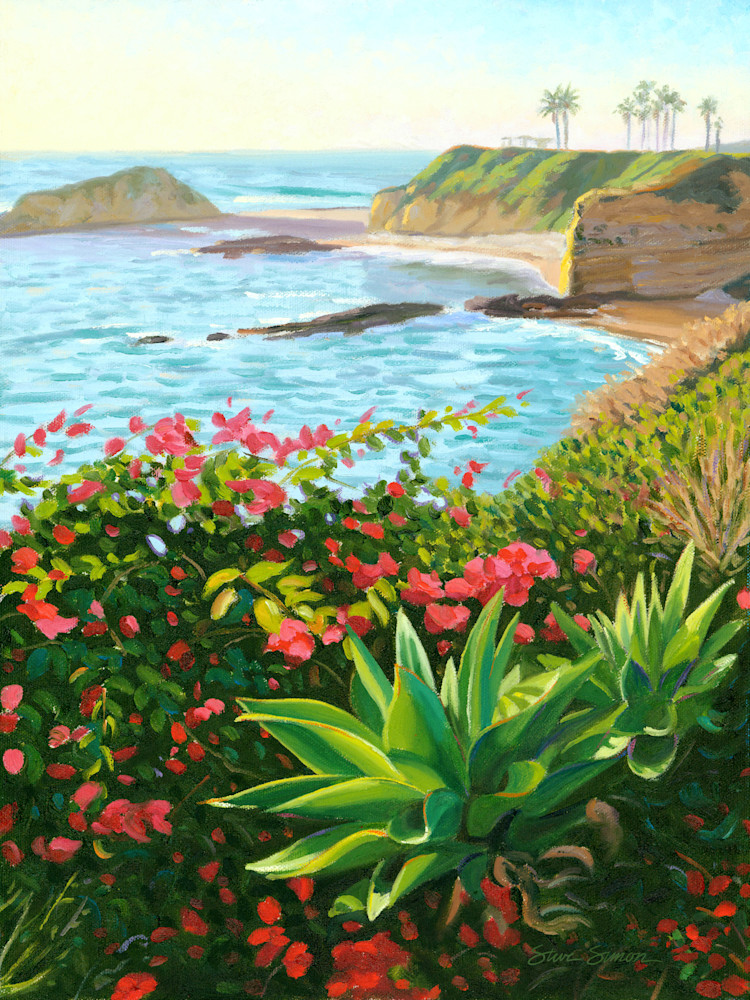This vibrant, tropical painting captures a serene coastal scene with meticulous detail. The foreground dominates with lush foliage, including two prominent bright green succulent plants that feature realistic shading and white highlights. These succulents are surrounded by a bush adorned with scattered red and pink flowers. The rocky shoreline stretches along the edge of the vivid blue ocean, where the water displays a mesmerizing ripple effect with shades of light blue, dark blue, and white. At the base of the rocks, green grass softens the transition to the sandy beach. A majestic cliff rises beside the beach, crowned with verdant green and dotted with palm trees reaching towards a sky that transitions from blue to a warm yellow hue near the horizon. Farther back, the ocean extends infinitely, evoking the sense of an idyllic lagoon or private retreat. The painting is signed by Steve Simon in the bottom right corner, further adding to its sense of artistry and personal touch.